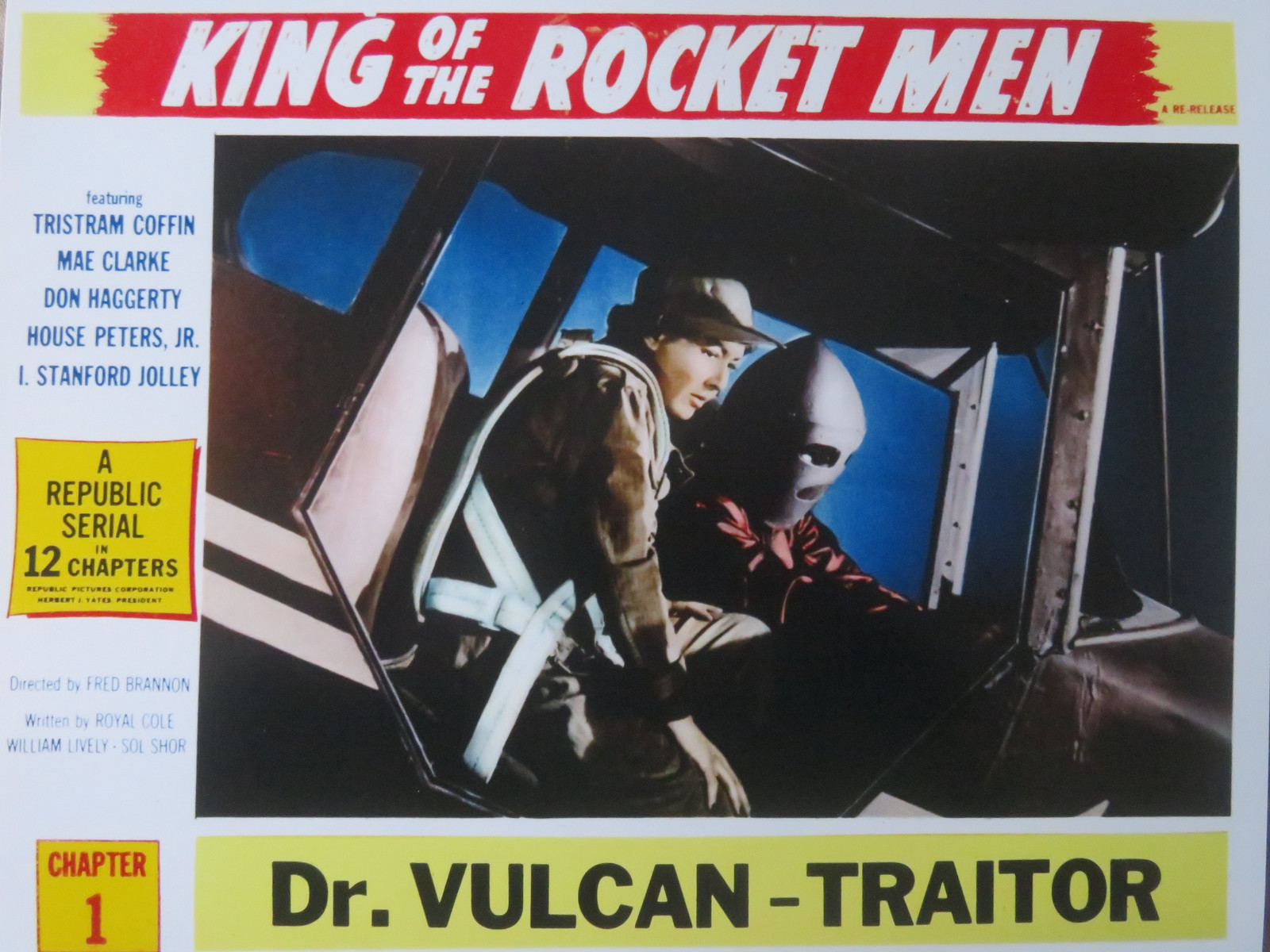The image appears to be a promotional poster for a vintage film or serial titled "King of the Rocket Men," highlighted in white with a bright red background at the top. Below the title is a prominent photo featuring two characters inside a sleek, metallic, doorless flying vessel. On the left is a woman, dressed in a brown jacket with white straps and a gray hat, while to her right is a man donned in a shiny, rocket-shaped helmet and a red jacket, reminiscent of military attire.

To the right of the photo, colorful text lists the cast and crew: "Featuring Tristram Coffin, May Clark, Don Haggerty, House Peters Jr., and I. Stanford Jolly." It also notes that it is a "Republic Serial in 12 chapters" produced by Republic Features Corporation with Herbert J. Yates as President, directed by Fred Brannan, and written by Royal Cole and William Lively. At the bottom in bold, black text, it reads "Dr. Vulcan – Traitor," indicating that this is Chapter One of the serial. The overall design and vivid colors suggest a dynamic and adventurous narrative.